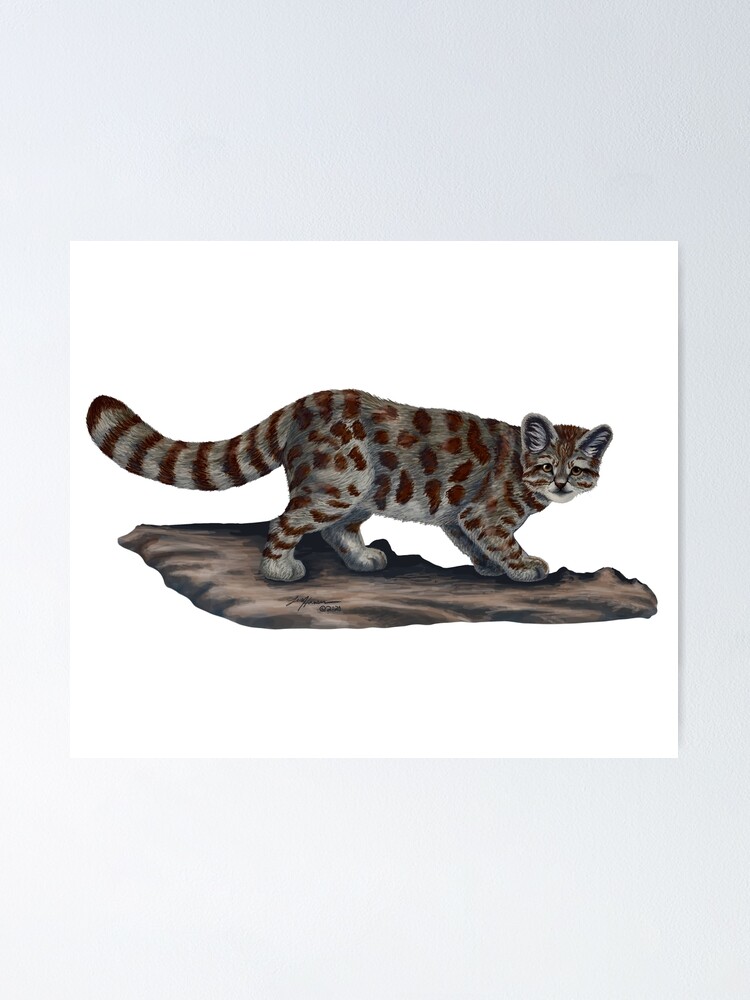The image depicts a detailed painting of a gray wild cat with rusty brown spots. The cat's unique tail features rings, reminiscent of a raccoon's tail. It’s crouching slightly, with its ears perked up, lined with white fur. The background of the image is predominantly white, suggesting that this might be a poster or artwork displayed on a white wall. The ground beneath the cat, also part of the artistic composition, is brown. The artist's signature is visible on the ground, adding an extra touch of realism and ownership to this exquisite piece of art.